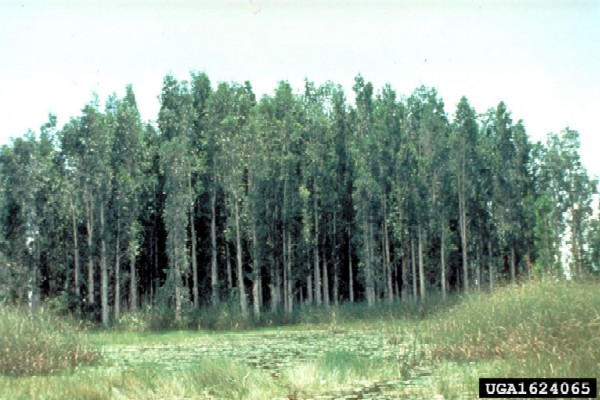The image depicts a dense cluster of tall green trees under a white or light blue sky, suggesting a lush, summery scene. In the foreground, there's a grassy field interspersed with patches of taller grass on the left and right, featuring flecks of yellow amidst the green. The trees are closely packed, creating a dark, almost black appearance where their canopies overlap. Some low bushes and scattered grassy areas populate the field in front of the trees. A black rectangle in the bottom right corner displays the text "UGA L1624065," adding a distinct label to the scene. The overall impression is of a serene, natural landscape dominated by the thick foliage of the trees.